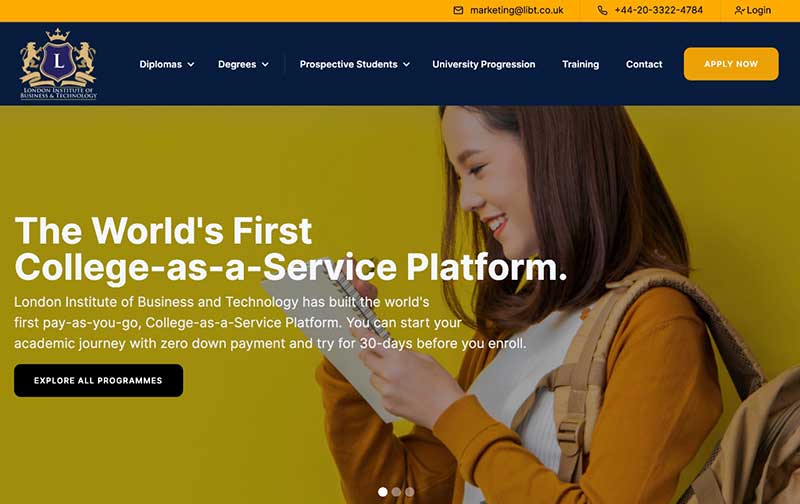This image is from the website of the Lincoln Institute of Business and Technology. In the upper left corner, there is a detailed logo featuring two gold lions standing on either side of a shield, adorned with a gold crown on top and ribbons below. The shield prominently displays an 'L'. 

In the website's navigation bar, tabs for various sections such as Diplomas, Degrees, Prospective Students, University Progression, Training, and Contact are visible, along with an "Apply Now" button. At the top of the page, the contact information is listed, including an email address (marketing@libt.co.uk) and a phone number.

The main focal point of the image is a photograph of a young, happy Asian student with a bright smile and red lipstick, her top teeth visible. The accompanying text reads, "The world's first college as a service platform. The London Institute of Business and Technology has built the world's first pay-as-you-go college as a service platform. You can start your academic journey with us."